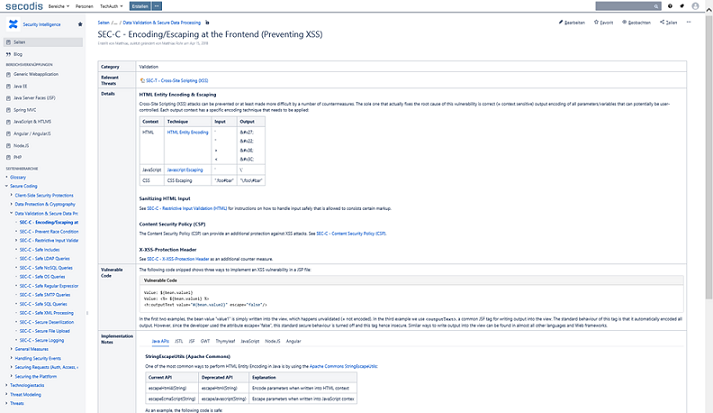A blurry and hard-to-read webpage displays a header at the upper left with the text "Seqotus." Below this, there are some illegible writings and a list on the left side of the page, which is also unreadable. At the top right, the text "sec-c-encoding-escaping-at-the-front-end" is visible, followed by the phrase "(preventing XSS)" in parentheses. Beneath this header, there is a body of text that could potentially be from a wiki page, though it is unclear. A table is present on the page with a column labeled "Category," which appears to be about "Validation," though the exact details are difficult to discern due to the blurriness. Various headings and sections are distributed throughout the page, but their content is indecipherable.